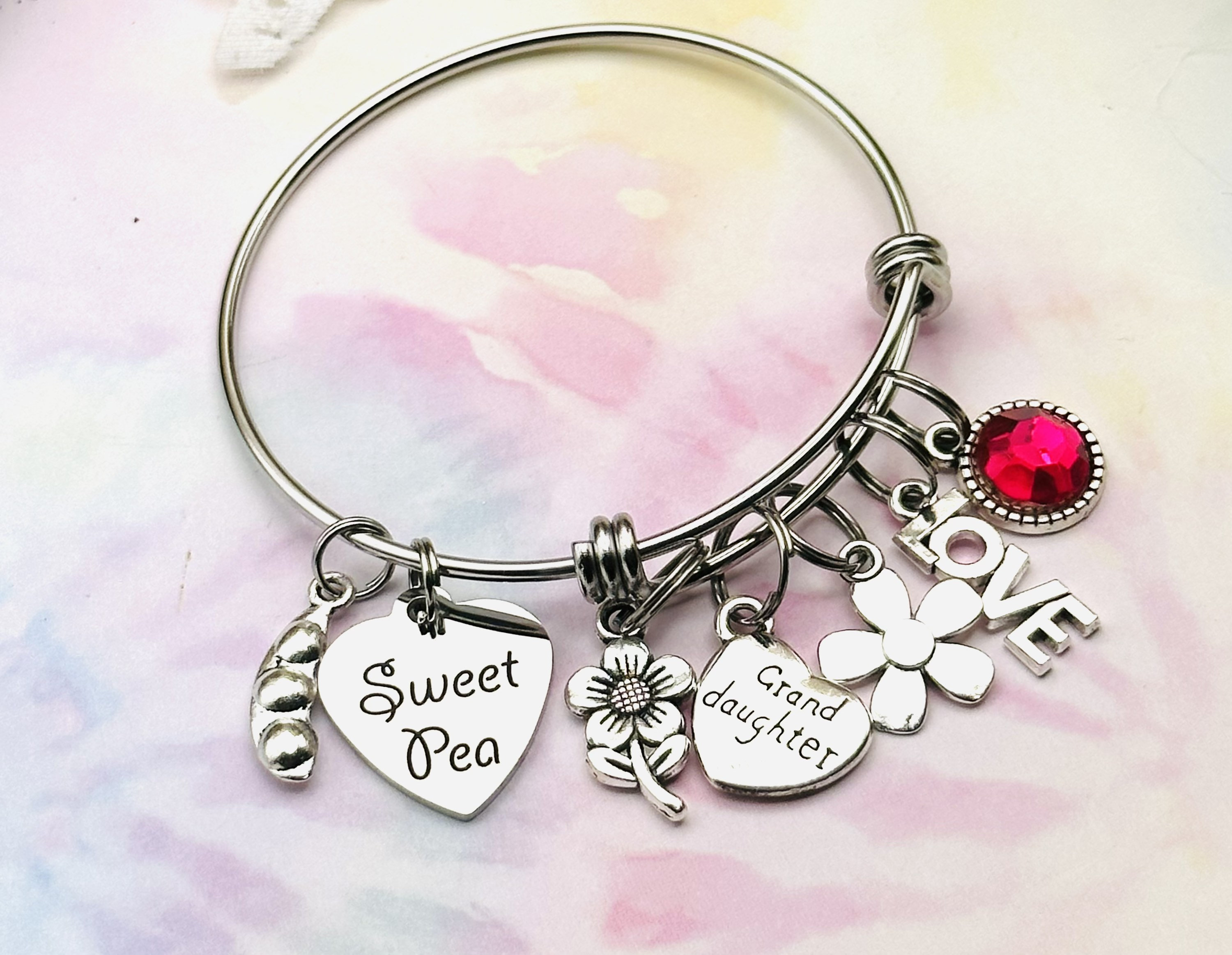This close-up photograph captures an intricate silver charm bracelet laid out on a table with a multicolored, pastel abstract watercolor backdrop of yellow, pink, and blue hues. The bracelet, approximately three and a half inches in diameter, features seven polished silver charms. The first charm depicts a pod with two peas, complete with circular ridges. The second charm is a heart inscribed with “Sweet Pea.” The third charm is a five-petal flower. The fourth charm is another heart, this one engraved with “Granddaughter.” The fifth charm is a plain five-petal flower. The sixth charm is made up of the letters “L-O-V-E” in silver. The final charm is a round pendant featuring a ruby-like gemstone. The overall composition of the photograph delicately balances the intricacy of the bracelet and the charm details against the softly marbled, pastel-colored background.